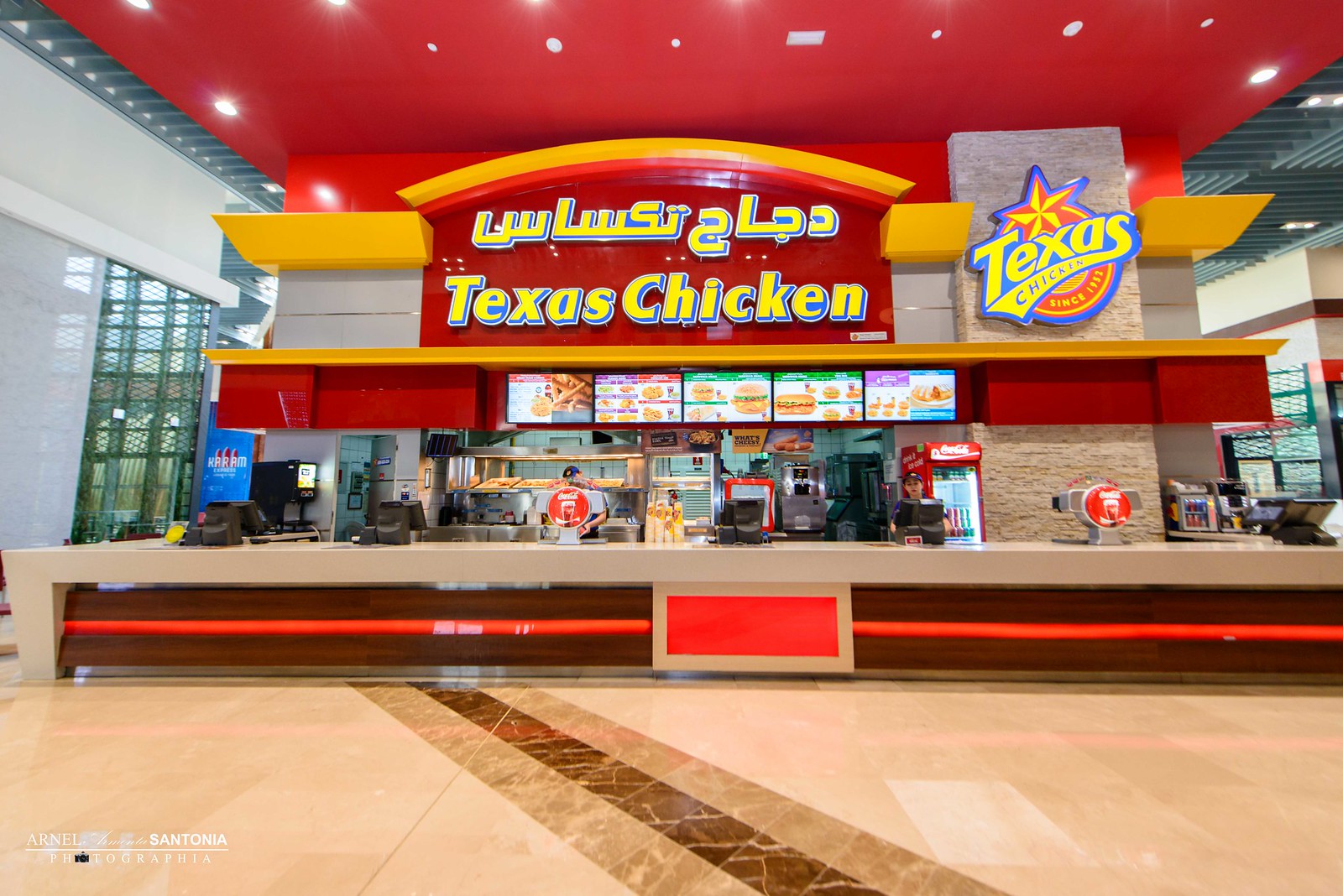The image captures the interior of a Texas Chicken fast food restaurant located within a larger building, likely a mall. The storefront features a prominent red sign that reads "Texas Chicken" in English, with additional text in a different language above it. To the right, there's a circular logo displaying "Texas Chicken" in yellow font with a blue border, accompanied by a red and yellow star. The counter where customers place their orders is characterized by a wood grain base embellished with a vibrant red stripe. The countertop itself is a pristine white marble-like surface. Behind the counter, staff members in blue uniforms can be seen, one attending to a Coca-Cola beverage machine, and another at the register. The menu is displayed on five different screens showcasing chicken sandwiches, various sides, and drinks. The flooring in front of the counter is made of beige marble with lighter tan and brown streaks. The restaurant setup suggests it's part of a food court, maintaining a functional design without seating areas.